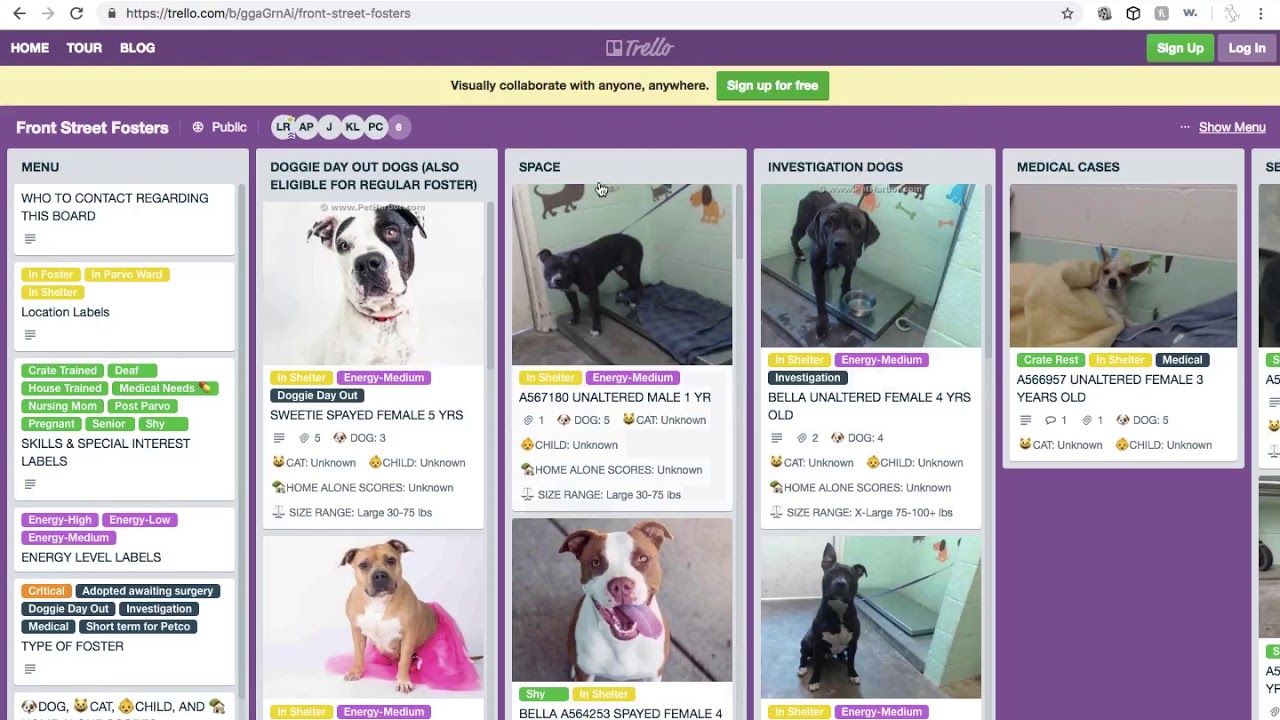The image portrays a webpage from Trello, indicated by the URL at the top. A prominent purple banner displays the text "Home Tour Blog" alongside the Trello logo, with options to sign up or log in. Below, a pale yellow strip features a call to action: "Visually collaborate with anyone anywhere," accompanied by a green "Sign Up for Free" button.

Central to the page is the "Front Street Fosters" board, marked as public and actively accessed by various users. A menu on the left-hand side provides options for connecting or contacting board members, categorized with yellow location labels. Below, green tabs detail specific needs and conditions of the dogs, such as "great," "trained," "deaf," "house trained," "medical needs," "nursing mom," "post parvo," "pregnant," "senior," and "shy." Purple labels indicate the dogs' energy levels.

The board also includes buttons for different types of foster care and features images of various dogs sorted into categories, such as "Doggy Day Out" dogs, regular fosters, and specific dogs like a sweet, spayed, five-year-old female, and an unaltered male, one year old. There are even sections for investigation dogs, providing users with an opportunity to click on each dog to learn more about them.